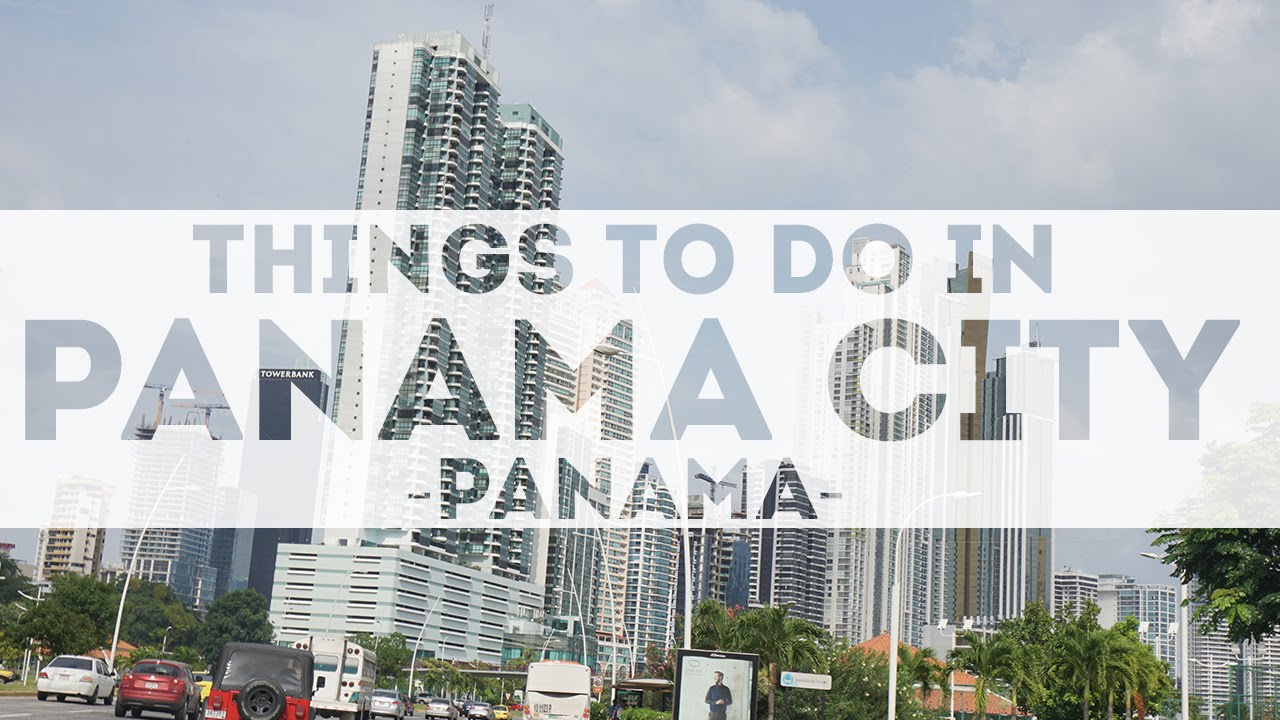The image captures a bustling city skyline dominated by towering condominium buildings reaching towards a partially cloudy sky painted in shades of light blue and white. In the foreground, a busy street teeming with traffic adds a dynamic element to the composition. A variety of vehicles populate the scene, including a red Jeep with black vinyl coverings, a red SUV, a white car displaying its red taillights, and the rear end of a white school bus. Additionally, a large commuter bus occupies a spot near the roadside. 

Skirting the borders of the image, one notices verdant palm trees standing adjacent to lower-rise buildings, one of which sports a distinctive slanted orange roof. Adding a human element, the bottom center features the silhouette of a man, outlined in black, as if depicted on the back of a bus stop sign. 

Overlaying this intricate scene is a stylish watermark, which reads "THINGS TO DO IN PANAMA CITY, PANAMA" in all capital letters. The text is set against a faded white rectangle that is completely transparent, allowing the vibrant cityscape to shine through each letter. 

The overall ambiance created by this combination of architectural grandeur, urban activity, and natural beauty, all under a sky tinged with the promise of varying weather, encapsulates the lively essence of Panama City, Panama.